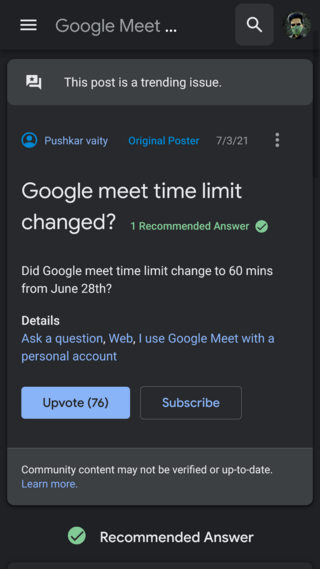A user is viewing a Google Meet help page. The central focus is a notification indicating a change in the Google Meet time limit to 60 minutes, effective from June 28th. Beneath this notification, there's a section for user questions, highlighting one particular inquiry with a green checkmark next to a "Recommended Answer" tag. The question is about using Google Meet with a personal account and has received 76 upvotes, signifying community agreement.

The display includes a blue-highlighted question and a black "Subscribe" button. Below it, in a lighter gray box, is a disclaimer stating, "Community content may not be verified or up-to-date." There's also a "Learn More" button underlined with a green checkmark, indicating a redundant recommendation.

The original query was posted by a user named Pushkar on July 3rd, 2021. The details about the upvotes signify community endorsement, making it easier for users to identify credible solutions. At the top left of the screen are the settings options, followed by "Google Meet..." and a search bar. To the right, the user's avatar, resembling a Mortal Kombat character with a green mask, indicates the logged-in user's identity.